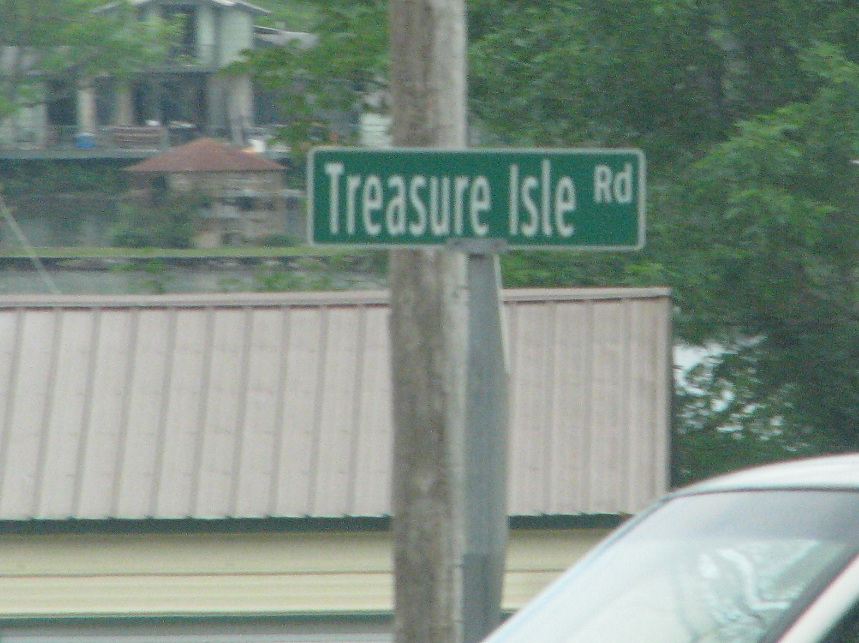The photograph captures a street scene dominated by a rectangular street sign with a green background and white text that reads "Treasure Island Road." Positioned prominently in the foreground, the sign is supported by a metal pole. Directly behind the street sign, a tree trunk rises, partially obscuring a view of a large metallic wall or fence.

In the background, abundant foliage is visible, with multiple trees laden with leaves framing the scene. To the left, part of a substantial house can be seen in the distance, characterized by its size and structure. In front of this house is a smaller building, possibly a shed, featuring a triangular roof with a reddish hue.

Additionally, the bottom right corner of the image includes an interior glimpse of a white car, specifically its windshield and upper dashboard, suggesting that the photo was taken from inside the vehicle.